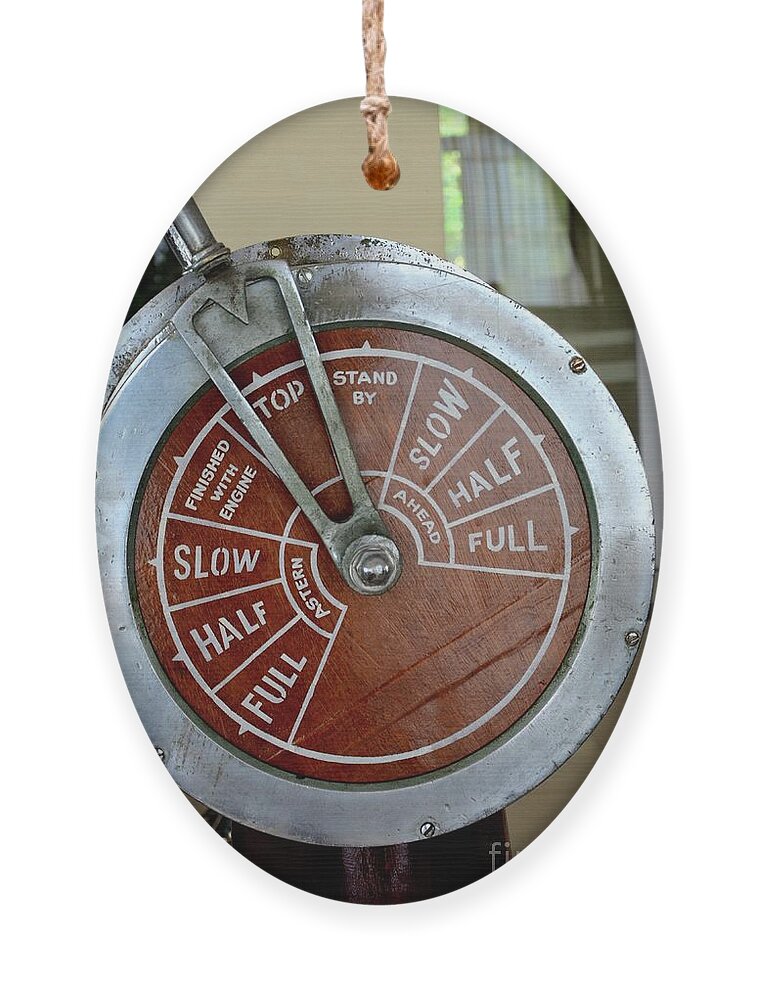The image showcases a detailed view of a ship's engine order telegraph, a crucial instrument used by the captain to control the ship's speed. This metallic device features a central dial encircled by various speed settings labeled in white, including "Full," "Half," "Slow," "Finished with Engine," "Top," "Standby," and "Stop." The dial is divided into two main sections: the left side marked "Astern" (indicating reverse) and the right side marked "Ahead." The lever on this dial can be moved to the desired speed setting, allowing precise control over the vessel's propulsion.

The device is presented in an oval-style image, with a thin vertical rope seemingly suspending it. The telegraph itself has a brown circular interior, likely made of wood, which contrasts with its steel mechanical exterior. In the background, there are visible window blinds and a cream-colored wall, adding to the nautical ambiance. The detailed design of the telegraph, with its white points and bordered angles, highlights the importance and functionality of this essential maritime tool.